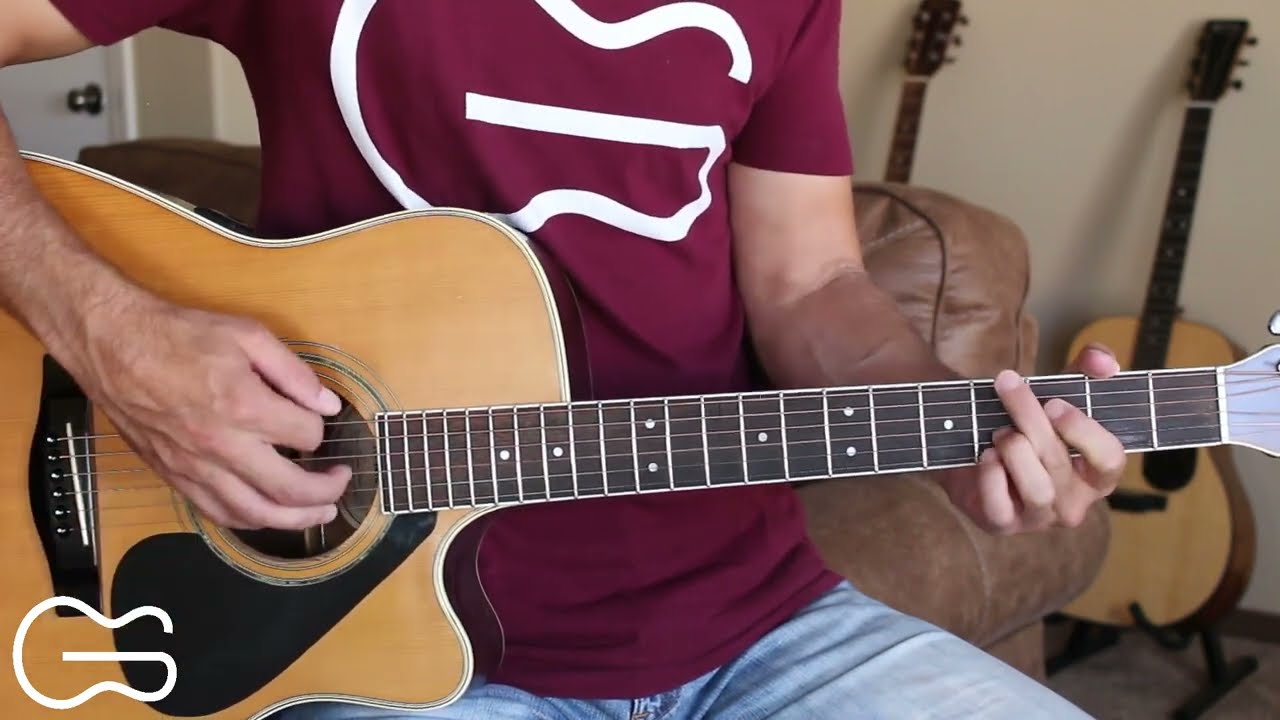The image captures a man seated on the edge of a brown leather or pleather chair in what appears to be a cozy living room. His face is out of view, and the image focuses primarily on his torso and the acoustic guitar he is playing. The man wears a red or burgundy t-shirt adorned with a white graphic design resembling the bottom of a guitar, accompanied by blue jeans. His left hand grips the frets, poised to play, while his right hand is set to strum.

In the background against a yellow or beige wall, two more acoustic guitars rest, leaning casually next to a white door with a silver handle. The same guitar-shaped graphic from his shirt is seen in the lower left corner of the image, potentially suggesting an advertisement for guitar lessons or a music-themed promotion. The overall scene exudes a warm, homely aesthetic, with the focus on the musical ambiance created by the man and his guitar.